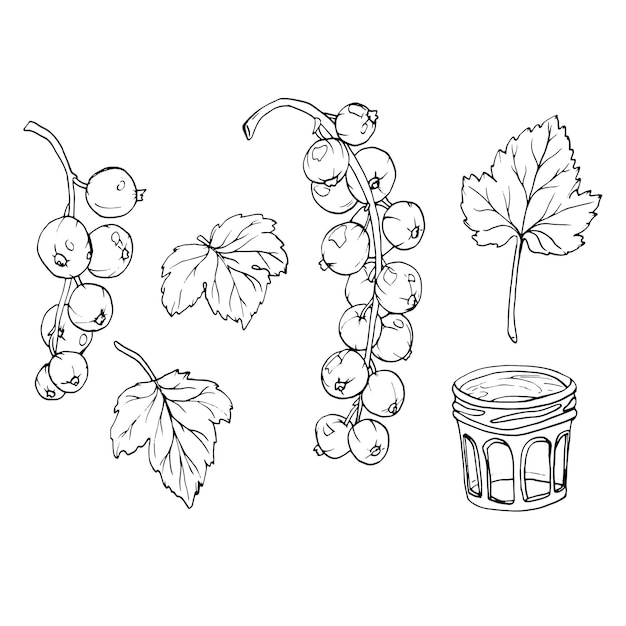This black and white, hand-drawn image, likely found in a book, features detailed and bold ink sketches on a white background. On the left, a curved stem showcases about seven blueberries hanging down. Adjacent to this are two distinct leaves: one with a long stem and another with a much shorter one, bearing a resemblance to Canadian maple leaves. In the middle-right, a longer, vertically oriented stem, curving from left to right, holds approximately 14 to 20 blueberries. The far-right portion of the image highlights another upright leaf with a lengthy stem and prominent veins. Below this, a round object resembling either a wastebasket or a drum, features arched window-like carvings encircling its entire surface. The composition is intricate, with high attention to detail in both the fruits and leaves.